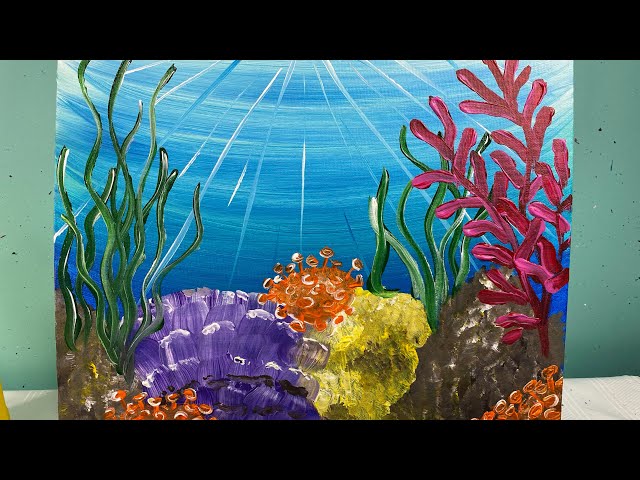This illustration depicts an underwater scene painted in a watercolor style. The background is a deep blue, reminiscent of ocean water, with beams of light penetrating from the top, illuminating the aquatic landscape below. On the left side, tall and wavy green plants extend from the bottom to the top, their leaves appearing to move with the water's flow. Among these, there are brown toadstool-like growths that resemble coral or rocks. Moving to the center, a peculiar orange object stands out with numerous lines that terminate in what look like suction cups, suggesting the vibrant variety of underwater flora. Surrounding this object are several other elements: a large purple object to the bottom left and another large orange entity. Further right, a yellow patch of brushwork depicts an additional piece of coral. On the far right side, a striking pink or purple plant with many leaves adds a splash of color to the scene. The bottom right corner features more orange coral-like structures accompanied by a gray section that may represent coral or rock. The overall composition captures the diversity and colorfulness of underwater plant life in a detailed and dynamic manner.